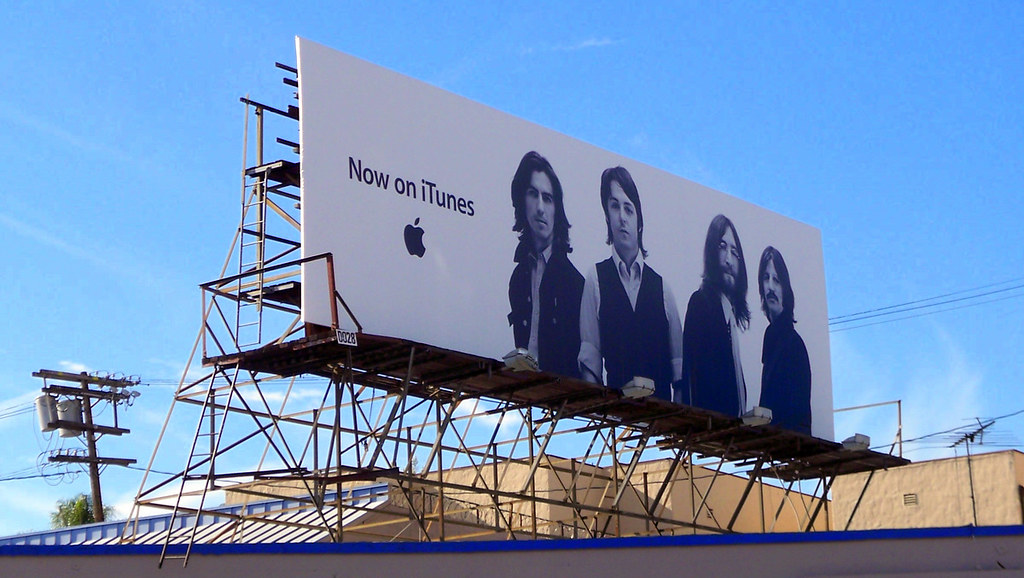A massive billboard, currently under construction with scaffolding and ladders visible along its sides, is prominently displayed high above beige stone buildings with slate roofs. This impressive billboard, supported by large iron posts, features a white background with the message "Now on iTunes" in bold black letters on the left beneath the iconic black Apple logo. The center of the billboard showcases a black-and-white image of The Beatles in their youth, dressed in their iconic fashion: Ringo Starr with a dark long-sleeved shirt and mustache, John Lennon with shoulder-length hair and a jacket over a white shirt, Paul McCartney with hair just below his ears in a rolled-up white shirt and dark vest, and George Harrison with shoulder-length hair, a light shirt, and a vest. The billboard is illuminated by several lights, and in the backdrop, a blue sky with a few wispy clouds is visible alongside telephone poles, electrical wires, and the tops of trees and buildings.